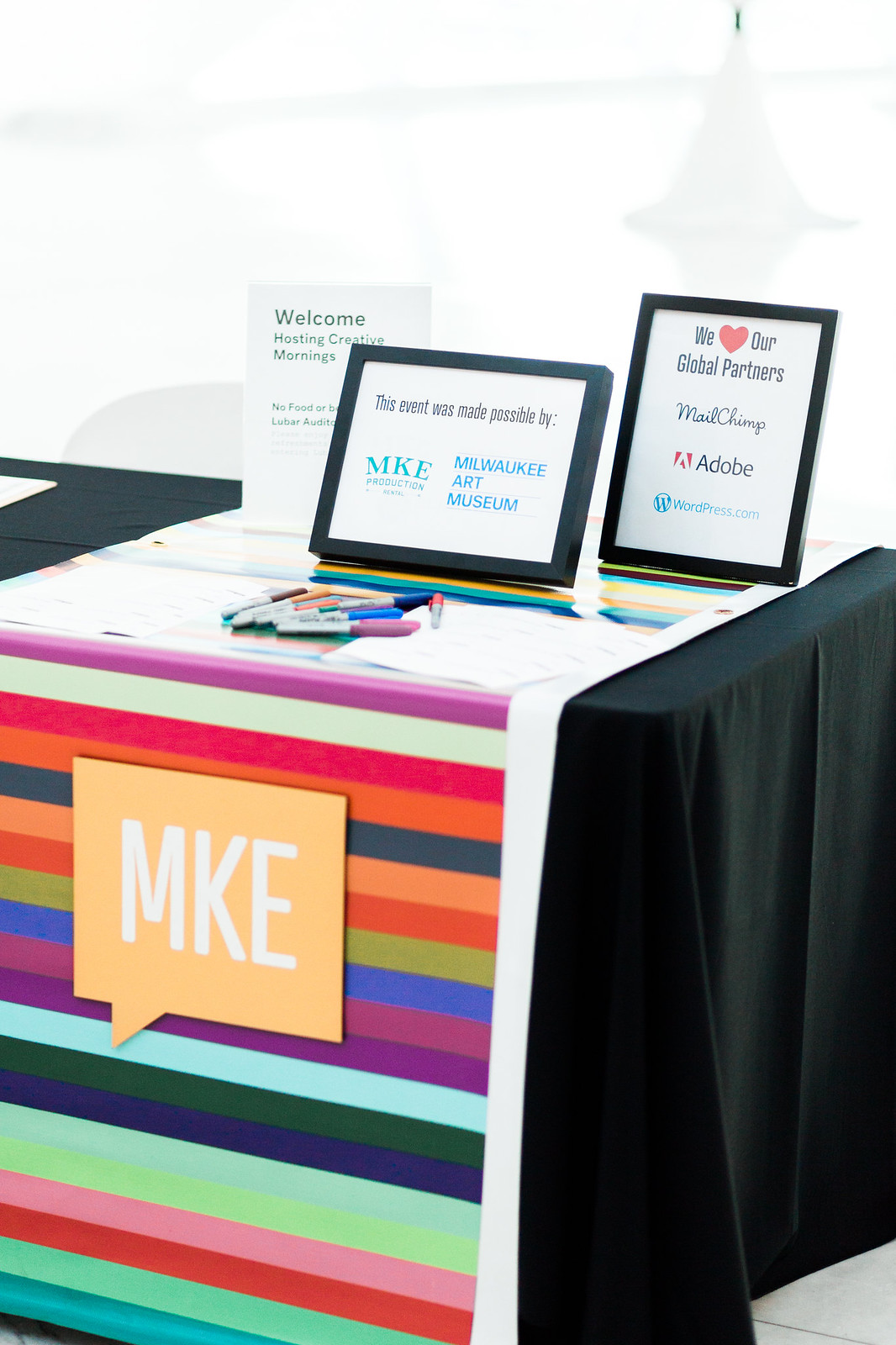This photograph captures a registration table likely set up for a conference or similar event. The table is draped with a black tablecloth, overlaid with a vibrant, rainbow-striped cloth that adds a splash of color. At the forefront of the table, there is a prominent orange-colored text box displaying the white letters "MKE." Various colored Sharpie markers are neatly arranged on the table, ready for use. There is a small welcome sign inviting attendees, and another sign that reads, "We love our global partners." Additionally, a third sign acknowledges the event's sponsor with the message, "This event was made possible by MKE Milwaukee Art Museum." The setup is both welcoming and informative, designed to make attendees feel appreciated and informed from the moment they arrive.